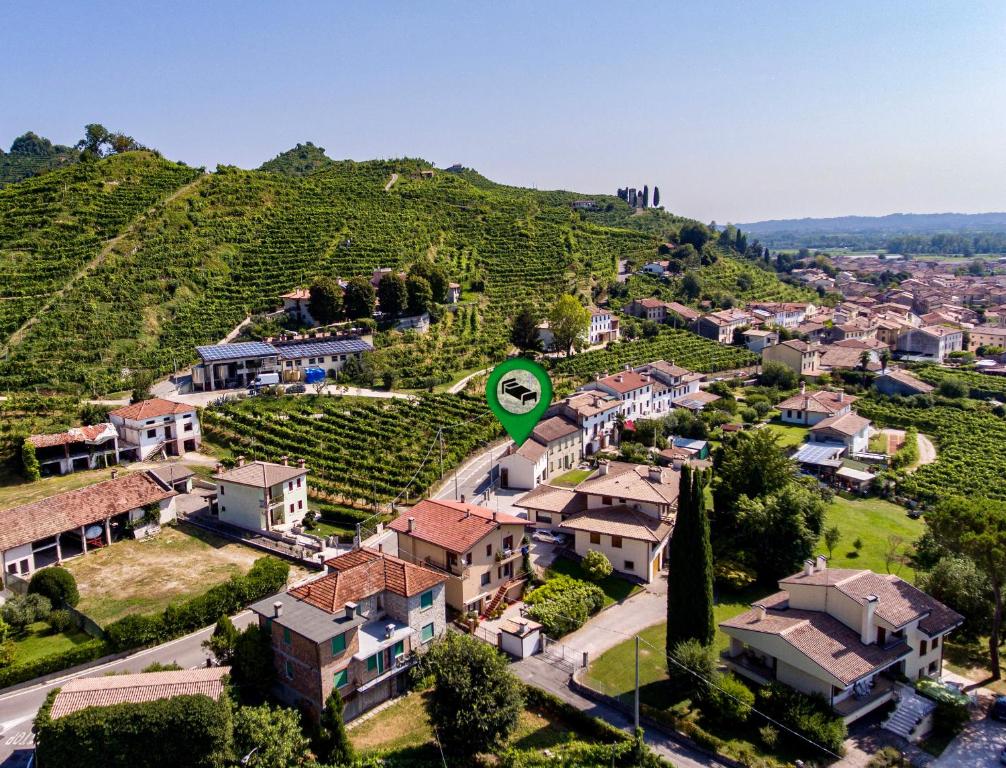This image is an aerial view of a verdant neighborhood situated on a large, grassy hill. Nestled amid the green expanse, which features wild-growing hedges and abundant trees, is a collection of buildings varying in size and color. Prominently, a green icon with a bed symbol suggests the presence of accommodations, possibly a motel or hotel, for visitors. A notable feature is a long, one-level building with a white van parked in front, alongside structures that could include a garage with open doors and a two-story white building. The houses, many with orange tile roofs, are spread throughout the landscape, which extends to a horizon dotted with trees and hints of a larger city in the distance. The scene is bathed in clear, blue sky, unmarred by clouds, and captures a tranquil, picturesque township seemingly ideal for a restful stay.